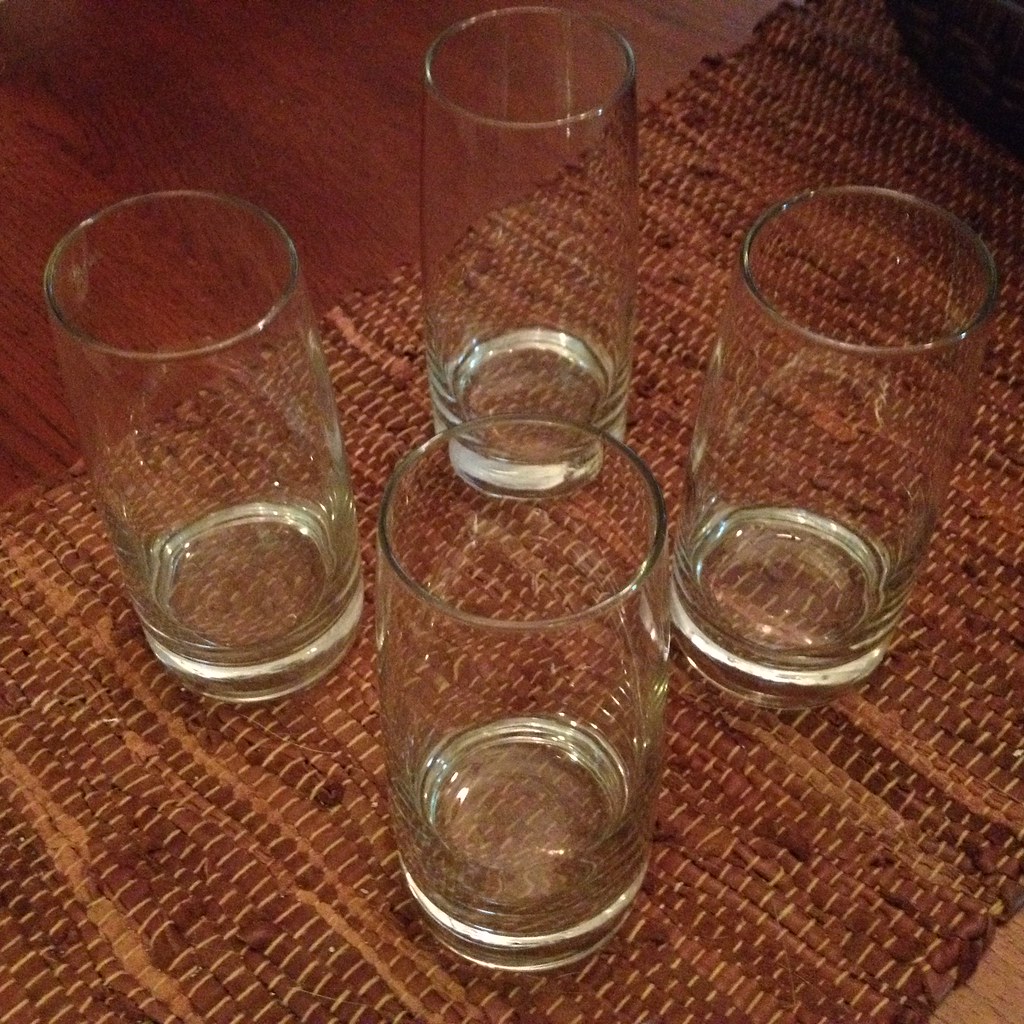This photograph features four tall, cylindrical glasses arranged in a diamond shape on a woven, red and white fabric mat. The mat, detailed with brownish-red and white stitching, sits atop a wooden table. The glasses, which are narrow with slightly rounded edges, are empty and reflect their surroundings, highlighting their glossy, freshly-cleaned appearance. The mat beneath them displays intricate knitted threads with dark brown rectangular areas and lighter brown threading interwoven. The clear glass allows the detailed fabric of the mat to be visible through them, presenting a simple yet aesthetically pleasing scene of neatly arranged glassware on a welcoming wooden surface.